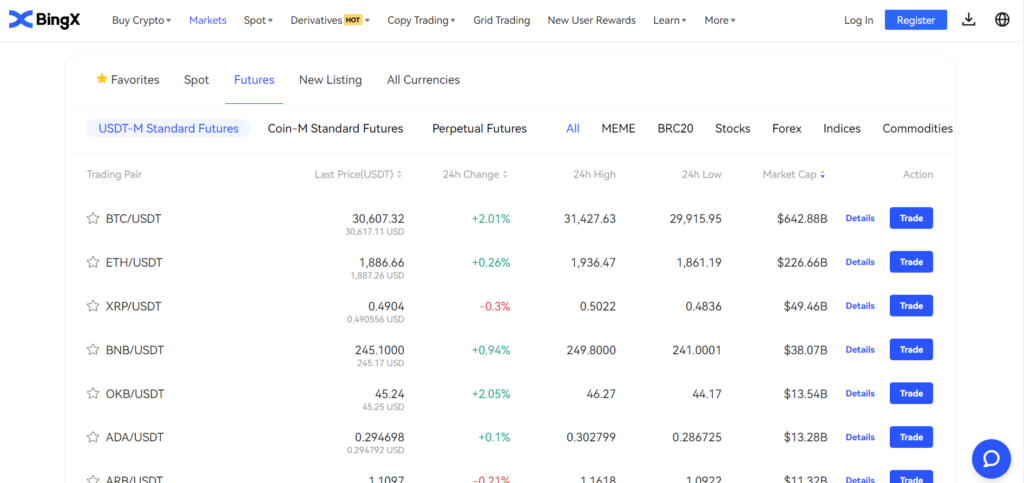The image displays a screenshot of a bank's website focused on cryptocurrency trading and various financial markets. At the top of the webpage, there is a navigation bar with options including "Buy Crypto," "Market," "Sport," "Derivatives," "Hard," "Copy Trading," "Grid Trading," "New User Rewards," "Learn," and more, alongside options to "Login" or "Register."

Below the navigation bar, there is a section promoting the website's "Favorite Sport Feature." This is followed by options to explore a "Search" function, "New Listing," and "All Currencies."

Further down, the page categorizes trading options into several groups: "USDT-M Standards Feature," "Coin-M Standard Feature," "Perpetual Futures," "All Meme," "BRC20," "Stocks," "Forex," "Indices," and "Commodities."

A detailed list of trading pairs is shown vertically, presenting combinations such as BTC/USDT, ETH/USDT, XRP/USDT, BNB/USDT, OKB/USDT, ADA/USDT, and others, with numerical data displayed alongside each pair, presumably representing current trading values or related statistics.